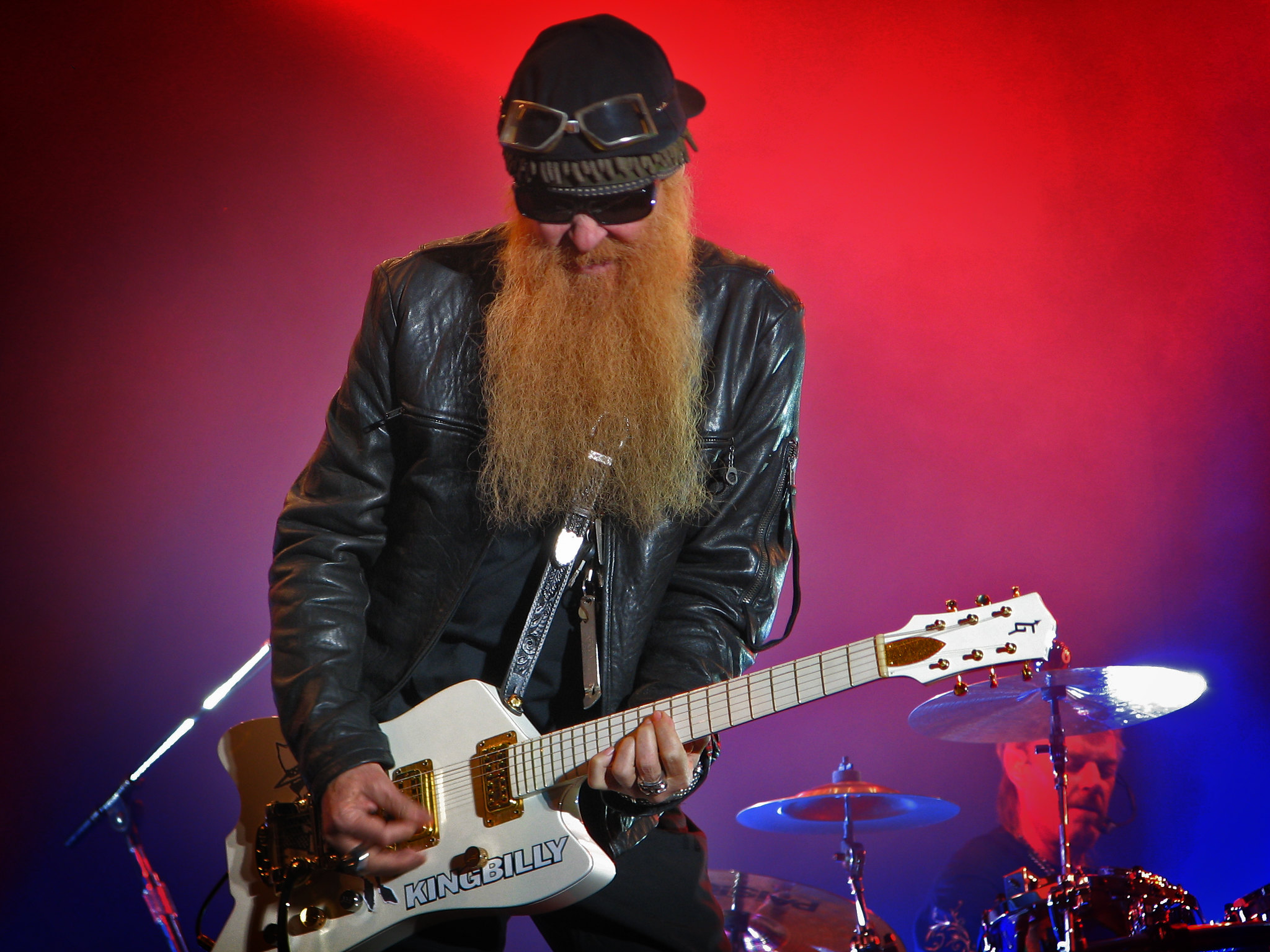In this image, a member of the legendary rock band ZZ Top is prominently featured mid-performance. The bearded guitarist, clad in a black leather jacket and black pants, sports a long brown or blonde beard, and wears a backwards hat adorned with goggles on top. He is also wearing dark sunglasses and multiple rings on both hands. Strapped across his shoulder is a striking white electric guitar with 'King Billy' emblazoned on it, accentuated by gold hardware and inputs. There is a backdrop suffused with red and blue hues, possibly from concert lighting or smoke effects, adding a vibrant atmosphere. Behind the guitarist, partially obscured by two cymbals, a drummer in a black t-shirt energetically plays the drums. The scene captures the electrifying energy of a ZZ Top performance, with the guitarist looking down at his instrument, deeply engrossed in the music.